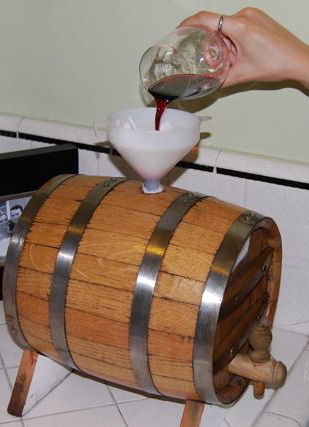In the detailed color photograph, a small wooden wine barrel, resembling a miniature cask, is the focal point. Adorned with four metal bands—two at the ends and two at the center—the barrel is positioned sideways on a sturdy wooden stand with white and wood-colored triangular bases at each end. A notable feature is a wooden spigot at the lower right front of the barrel. The top of the barrel, now on its side, has an inlet fitted with a white plastic funnel. From the top right of the image, a hand with a ring on the index finger holds a tipped-over wine glass, pouring dark red wine into the funnel. The scene is set on a white tiled countertop bordered by a black-rimmed white tile backsplash. Above it, the wall is painted a very light shade of green, providing a subtle backdrop. The image is captured in a portrait orientation, showcasing photographic representational realism.